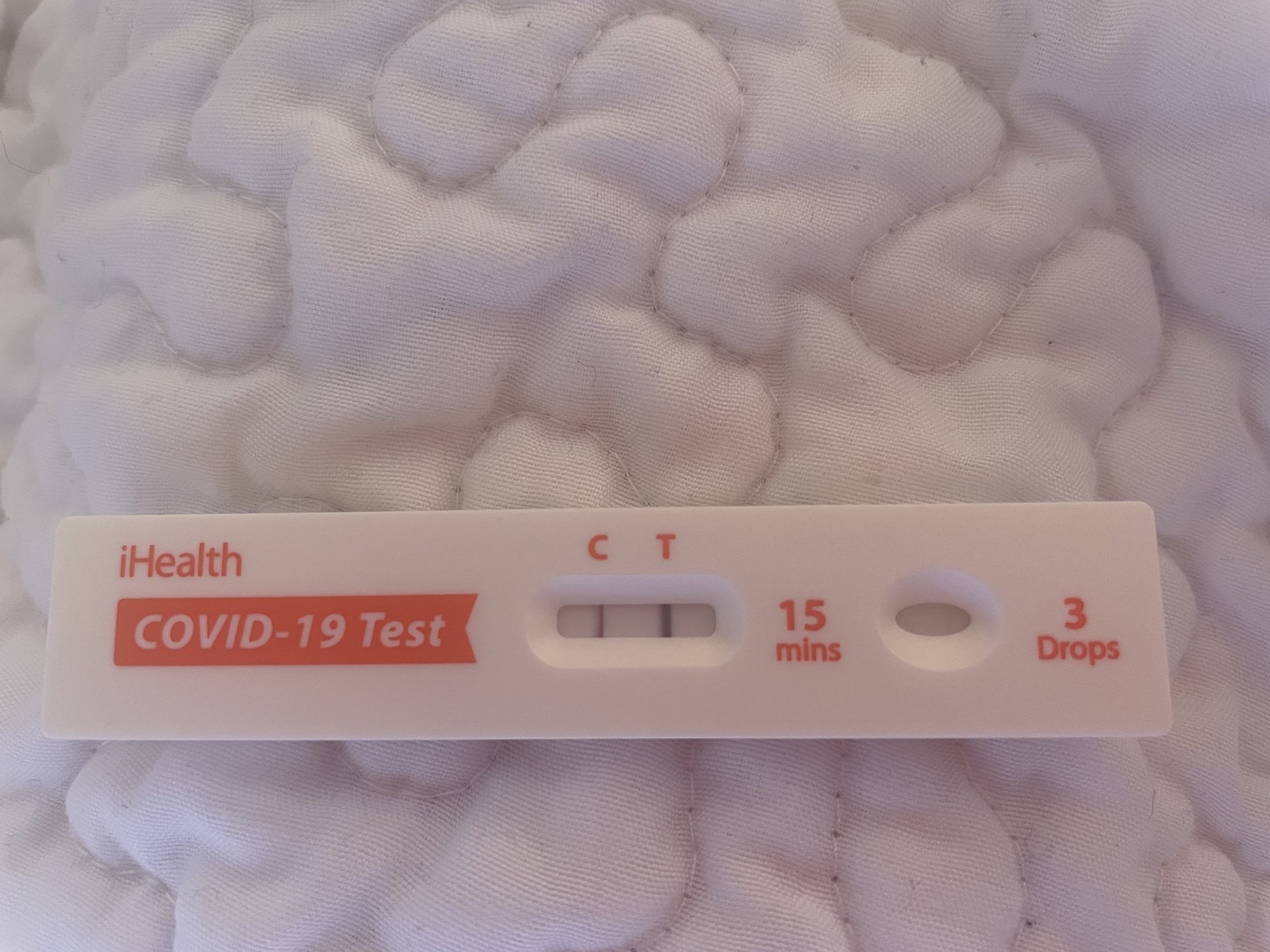A close-up image of an iHealth COVID-19 home test kit resting on a white, quilted blanket. The test strip, crafted from long, rectangular white plastic, prominently displays "iHealth" in white lettering on the left, followed by "COVID-19 test." Adjacent to this, there is a small window labeled with the letters "C" and "T", showing two lines beneath them to indicate the test result. To the right, it instructs "15 minutes" while another small window next to it is marked "3 drops," indicating where to deposit the testing fluid. The quilted blanket beneath the test strip has a soft, puffy texture, highlighted by needle quilting throughout. The intricate texture of the blanket contrasts gently with the smooth and clinical appearance of the test kit.